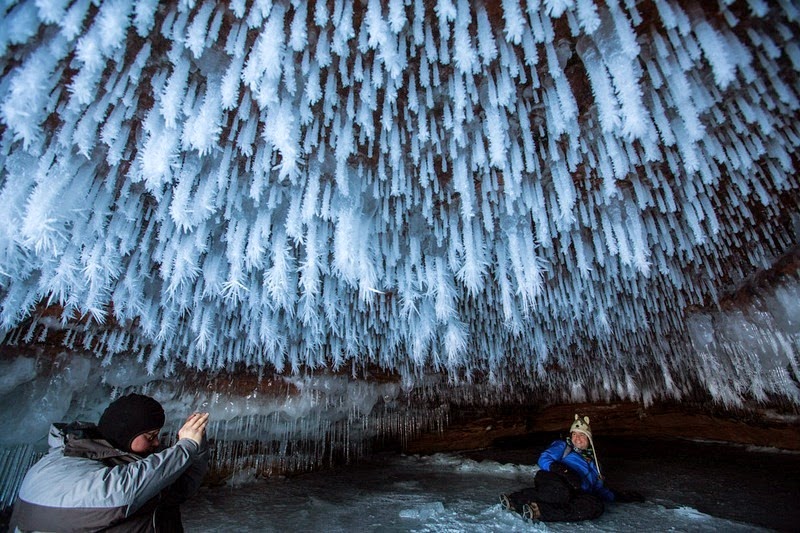In the foreground of the image, a man wearing a black hat and a large parka is holding up a camera, seemingly taking a photograph. In front of him, a person lies on the snowy ground, dressed in a blue coat, black pants, and brown boots. This person is smiling and wears a hat designed to look like a husky dog. They pose comfortably as the man captures their picture. The scene is set in an ice cave, evident by the numerous thick, frosted stalactites and icicles covering the ceiling above and the walls around them. The ice formations are intricate, with sharp, varied shapes, giving the cave a very cold, almost surreal appearance.